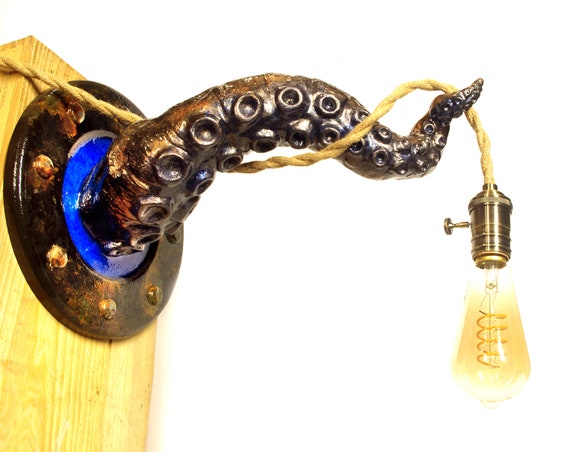This detailed photograph showcases a highly artistic lamp with multiple unique elements. The central focus is a vintage-style light bulb, featuring a toggle switch, suspended at the end of an intertwining electrical cord. The cord threads through and out of an elaborate, dark metal (possibly brass or copper) sculpture shaped like an octopus tentacle. This tentacle seems to reach out from the wall, complete with meticulously crafted suckers, giving it a lifelike appearance. The tentacle is anchored to a wooden pillar on the left side of the image, affixed with a metal plate and visible screws. Intriguingly, the core of this metal plate houses a vivid blue disc, adding a striking contrast to the dark, brassy hues of the tentacle and the otherwise neutral background, which is plain white.